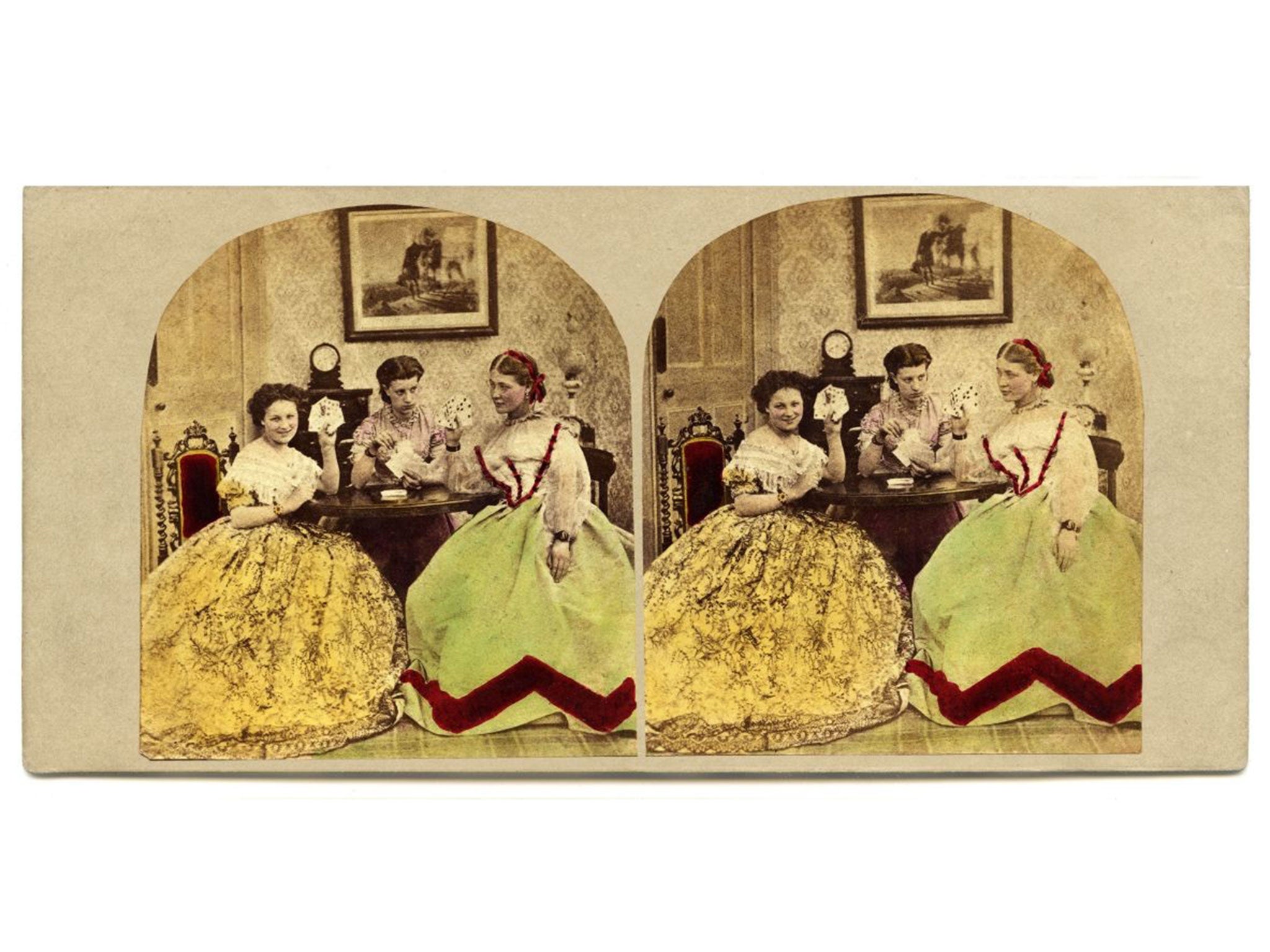The image is a wide-angle photograph featuring two identical sepia-toned pictures side-by-side, from possibly the late 1800s to early 1900s. Each picture features three women seated around a circular table, with the two women in the foreground wearing elaborate, floor-length dresses—one with yellow flowers and the other in a pale green dress with a red zigzag pattern along the bottom. The third woman, depicted behind the table, wears what appears to be a pink top, and they are all engaged in a card game as they hold playing cards in their hands. The women sit in high-back, velvety chairs, while behind them, a wall adorned with wallpaper and a six-panel chair rail is visible. A clock sits on a cabinet, and a portrait of a man standing next to a horse hangs on the wall. The photos are black-and-white with color added post-capture, and the top of each photo is rounded, reminiscent of a slice of bread. One of the copies is slightly clearer in color than the other, adding a subtle nuance to the vintage tableau.